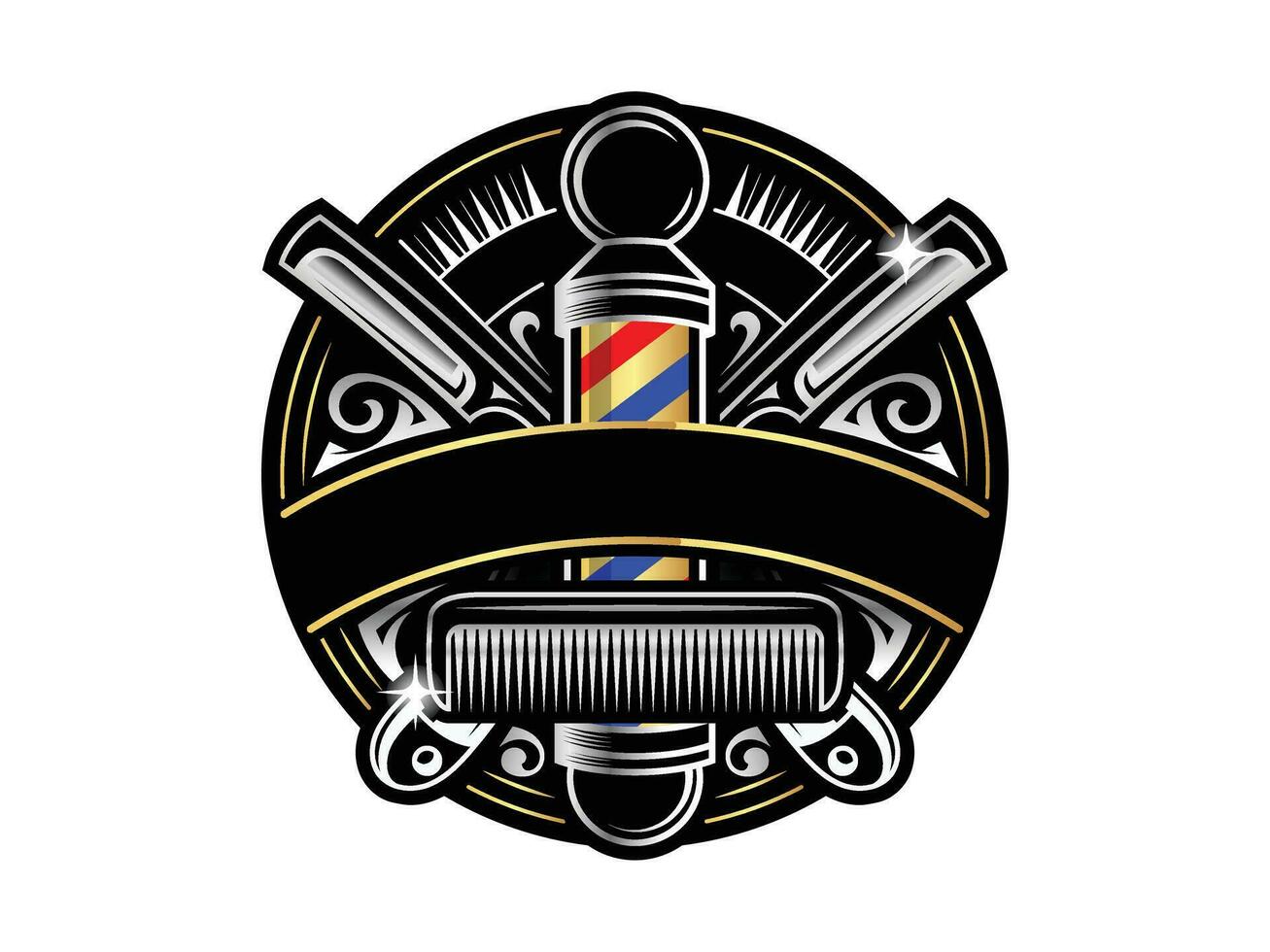This stylized barbershop logo is set against a round black background. Dominating the center is an old-fashioned barber pole with red, gold, and blue diagonal stripes running from the lower left to the upper right. Surrounding the pole are white outlines of classic barber tools including potentially old-style razors, scissors, and various combs. A prominent black comb with white teeth patterns is horizontally positioned in the foreground. Above the comb, a curved black banner with gold borders adds a decorative touch. Additional curlicues in white accent the design, creating a visually intricate and balanced composition reminiscent of vintage barbershop imagery. The colors black, gold, red, blue, and white feature prominently, giving the logo a classic and timeless feel. Despite its detailed elements, the design appears modern and is neatly contained within the circular frame, clearly representing a barbershop icon.